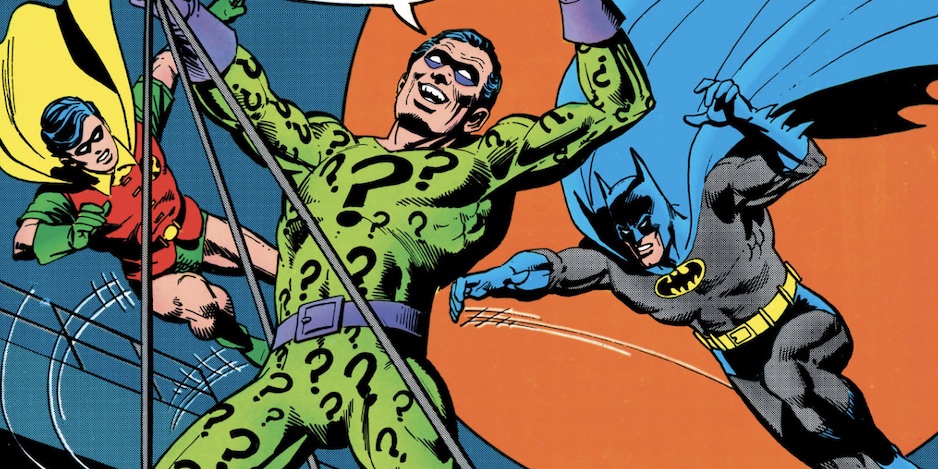This vibrant cartoon illustration from a DC comic strip features three iconic superheroes and a villain in a dynamic scene. On the left, Robin stands poised against a deep green background, wearing his distinctive red vest with a yellow 'R' near the chest, a yellow cape, green tights, green trunks, green gloves, and green boots. He appears to be reaching out and ready for action. In the center foreground, the Riddler takes the spotlight with his mischievous grin, dressed in a bright green bodysuit adorned with black question marks, a purple belt, blue hair, and blue goggles. He's tangled in a rope and appears to be attempting an escape. Hovering above his head is a speech bubble, but its contents are cut off. On the right side, Batman is captured mid-jump against an orange background, lunging towards the Riddler. He sports a blue cape, blue gloves, a grey suit with blue detailing, blue shorts, and a yellow belt. Prominently displayed on his chest is the iconic yellow and black Batman logo. This action-packed scene beautifully showcases the tension and drama of the superhero world.